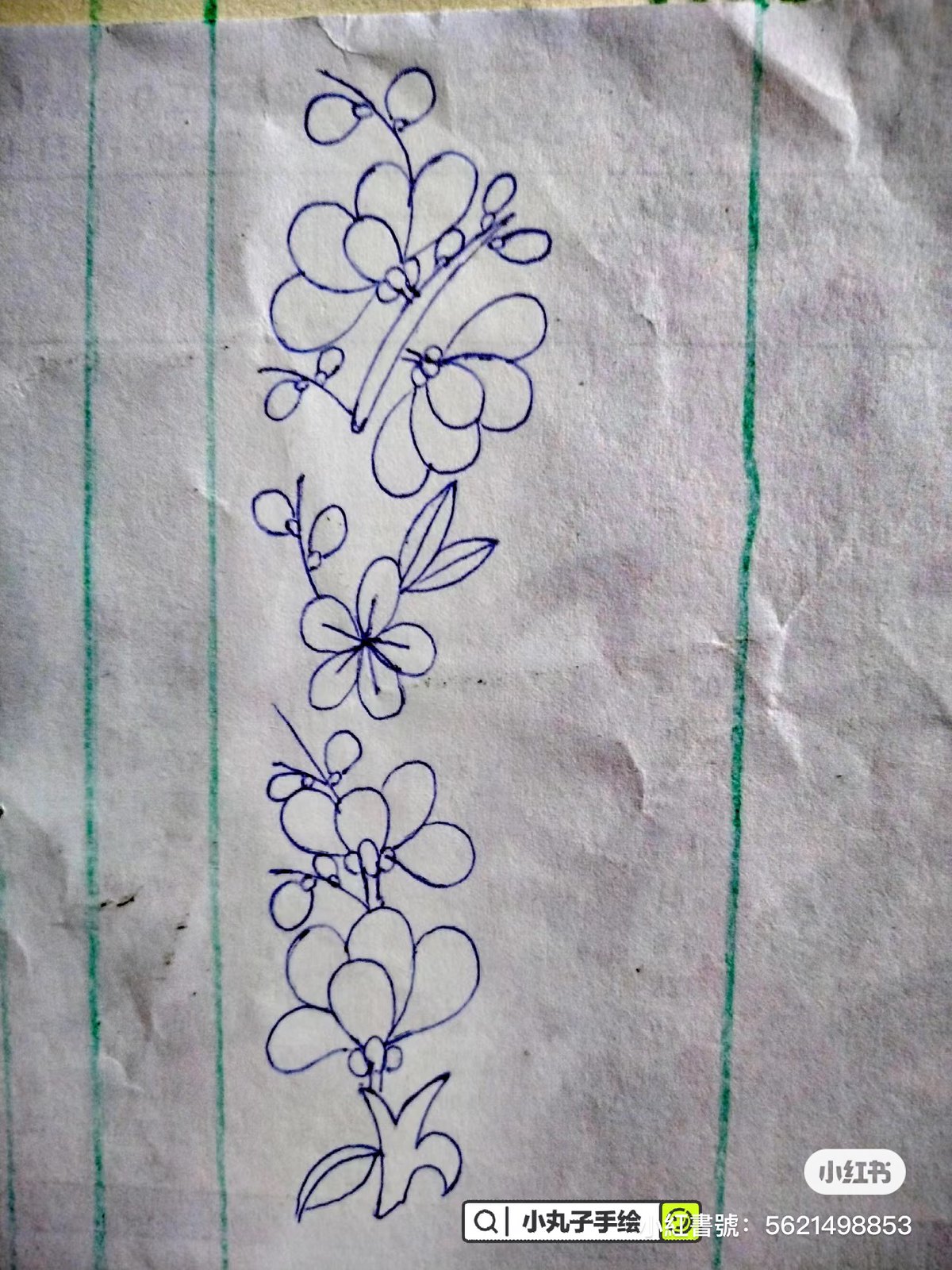This is a detailed pen drawing, executed in blue ink on notebook paper, depicting a cluster of flowers characteristic of the sakura (cherry blossom) species. The illustration is complemented by Japanese or Chinese text at the bottom, suggesting an East Asian cultural context. Although devoid of color, the drawing meticulously captures the intricate structure and delicate beauty of the blossoms, which are often celebrated during spring festivals in countries like Japan and Korea. The flowers are shown emerging gracefully from their branches, with some in full bloom and others just beginning to bud. This well-executed drawing, despite the lack of the iconic pink hue associated with sakura, is a charming piece that could easily serve as a design for a tattoo.